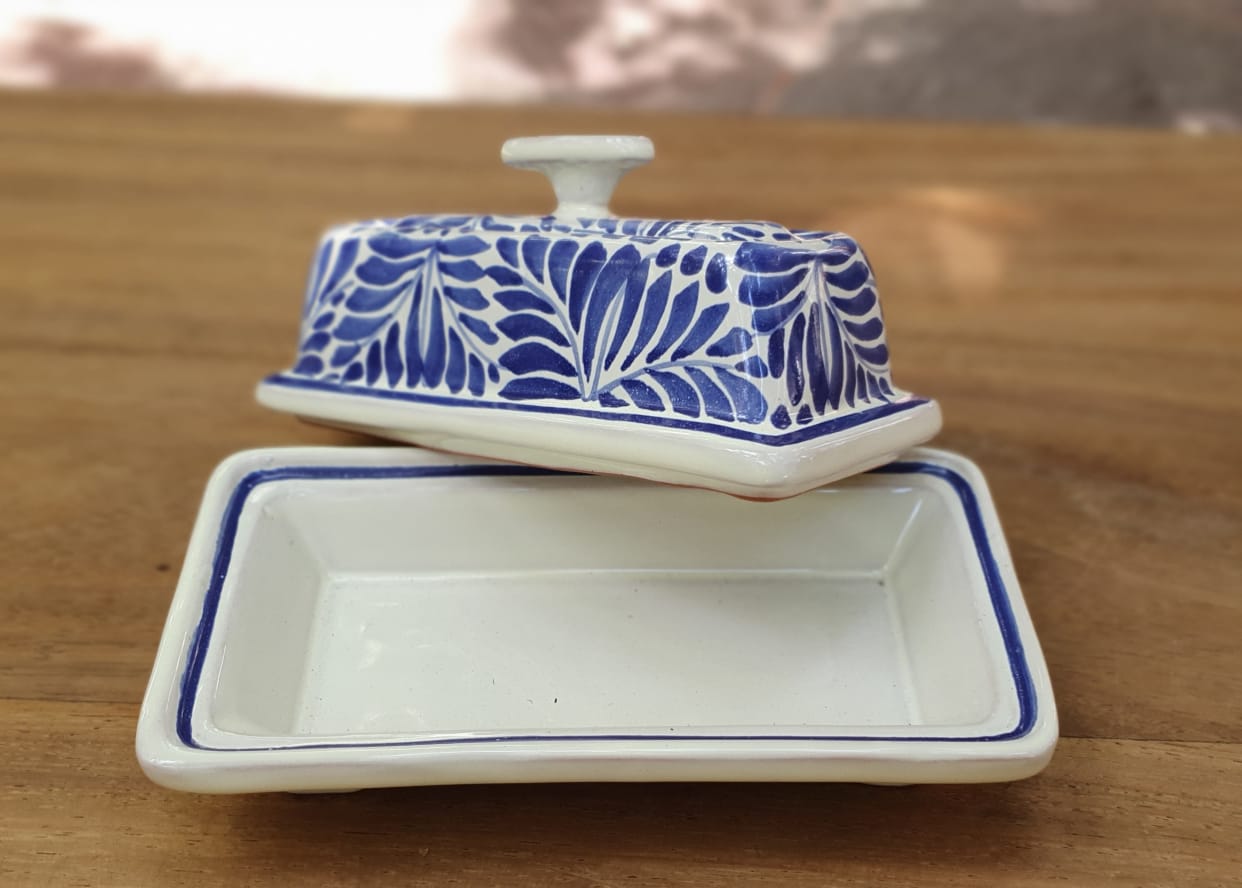The image depicts a horizontally aligned, rectangular ceramic butter dish placed on a large brown wooden table with natural wood coloration and visible horizontal grains. The scene appears to be outdoors under a dim sky, with blurry, hazy images of tree tops in the background. The butter dish is prominent in the foreground, with its lid partially off and positioned diagonally, half on the table and half on the dish. The dish's bottom half is predominantly white with a thin blue border, whereas the lid features a white handle and is adorned with a delicate leaf pattern consisting of light blue or gray stems and small dark blue leaves. This intricate design covers the top half of the lid, enhancing the overall aesthetic of the butter dish.